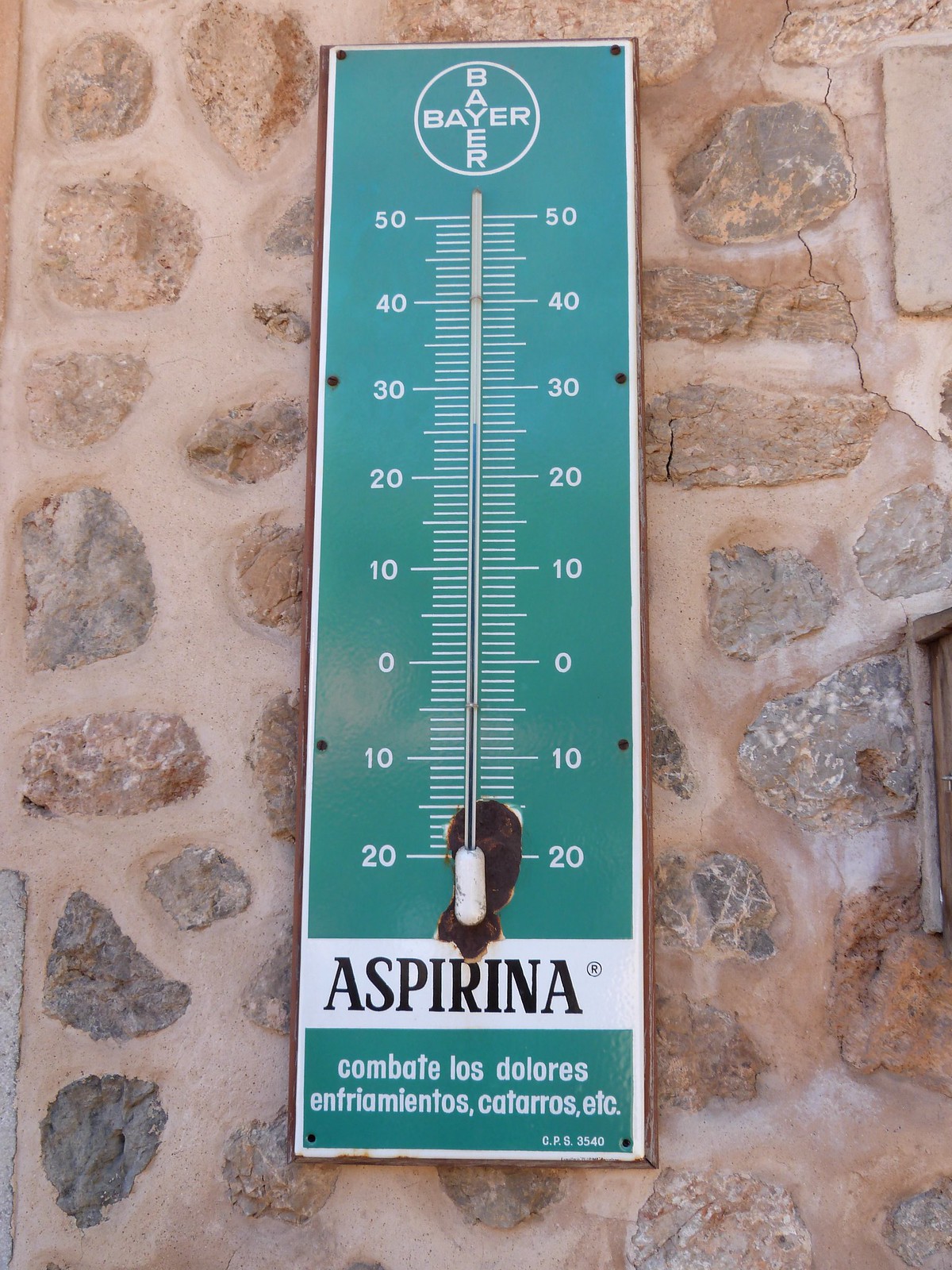Here's a detailed caption for the image:

"A Bayer-issued thermometer is securely mounted on a brick wall, precisely indicating a temperature of 26 degrees Celsius. The thermometer, designed entirely in the Celsius scale, features blue mercury and is notably attached to a light blue board with white lettering and numbering. At the top of the board, the brand name 'Bayer' is prominently displayed, while the bottom bears the word 'Esperina' in Spanish. The metal framework around the bulb of the thermometer exhibits significant rust. The rustic charm of the brick wall, which appears to be cobblestone, adds to the overall vintage aesthetic of the scene."